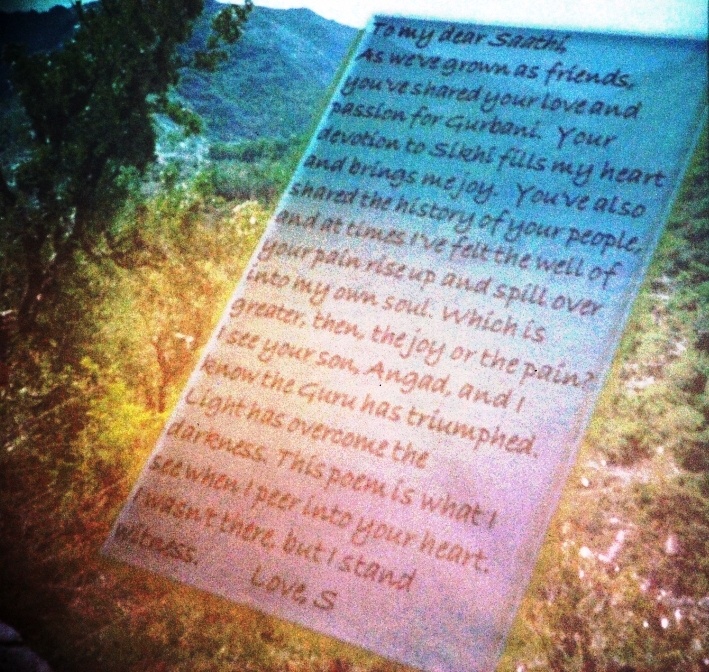The image is a grainy, textured collage featuring a treed landscape with hills and a heartfelt letter. The background is a colorful gradient with distinct sections: green vegetation on the side of a hill in the top left, transitioning to blue mountains and hills, followed by a yellow hue, red-brown tones in the lower left, and patches of white in the lower right. Overlaid on this vivid backdrop is a piece of paper with a gradient as well: blue at the top, white in the middle, and red at the bottom. The letter begins with "To my dear Sati," and expresses deep sentiments about friendship, love for Gurbani, and devotion to Sikhi. The writing shifts from black to red, culminating with the words, "This poem is what I see when I peer into your heart. I wasn't there, but I stand witness. Love, S."